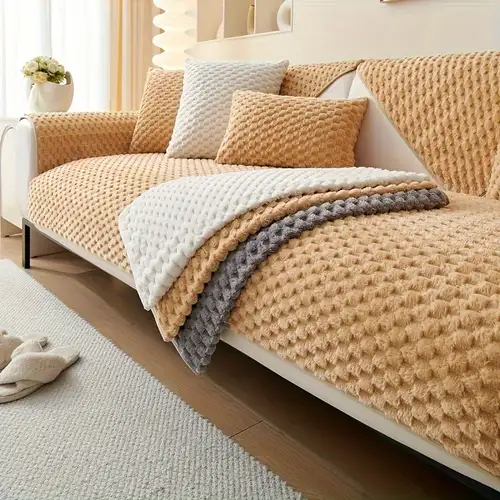This image captures a cozy, modern living room interior with a cream-colored couch adorned with a mustard-colored cover. The couch is positioned against a beige wall and features a variety of pillows: two tan pillows, one white pillow, and a mix of mustard, grayish-white, and white pillows for added comfort. A cushioned blanket in gray, white, mustard, and gray hues is draped over the side. 

On the floor, a white fluffy rug contrasts with the visible hardwood flooring beneath and a pair of cream-colored slippers rest on the rug’s surface. To the side of the couch, a white stand holds a ceramic vase containing a bouquet of white and yellow flowers with green leaves. 

The room is further complemented by off-white curtains, a shelving unit, and a cupboard that add to the modern aesthetic of the space. The overall minimalistic decor emphasizes a clean, spartan look, steering clear of any antique elements.